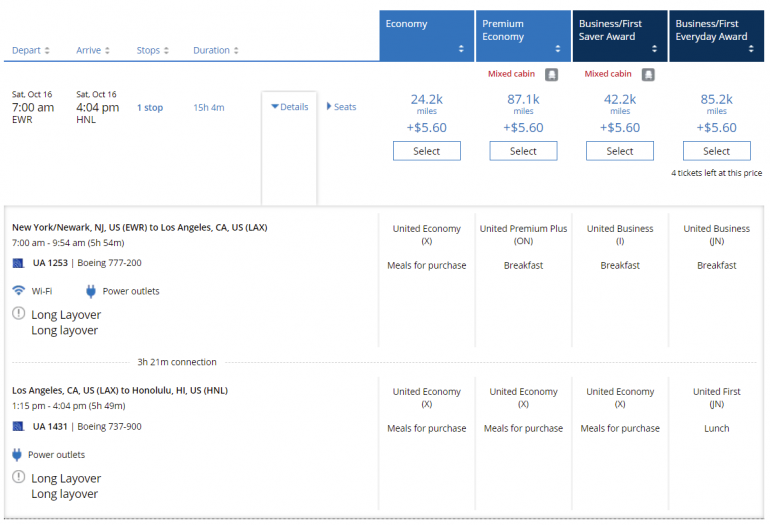This image is a screenshot of a flight booking web page. Positioned in the upper left-hand corner are drop-down menus labeled "Depart," "Arrive," "Stops," and "Duration." To the right of these menus are four tabs, indicating different travel classes: "Economy," "Premium Economy," "Business First Saver Award," and "Business First Everyday Award."

The selected flight details are displayed on the left side, under the heading bar. The itinerary shows a flight on Saturday, October 16th, departing at 7:00 a.m. from Newark Liberty International Airport (EWR) and arriving at 4:04 p.m. in Honolulu, Hawaii (HNL), with one stop. The total duration of the journey is 15 hours and 4 minutes. Adjacent to these details are price listings and "Select" buttons, indicating the number of miles required and associated costs.

Below this section, the specific flight legs are detailed. The first leg departs from Newark Liberty International Airport (EWR) in New Jersey, traveling to Los Angeles International Airport (LAX) in California. The second leg proceeds from Los Angeles (LAX) to Daniel K. Inouye International Airport (HNL) in Honolulu, Hawaii. Both legs indicate long layovers.

To the right of this flight information, meal options by travel class are listed: "United Economy" offers meals for purchase, "United Premium Plus" serves breakfast, "United Business" also serves breakfast, and "United First" includes lunch.